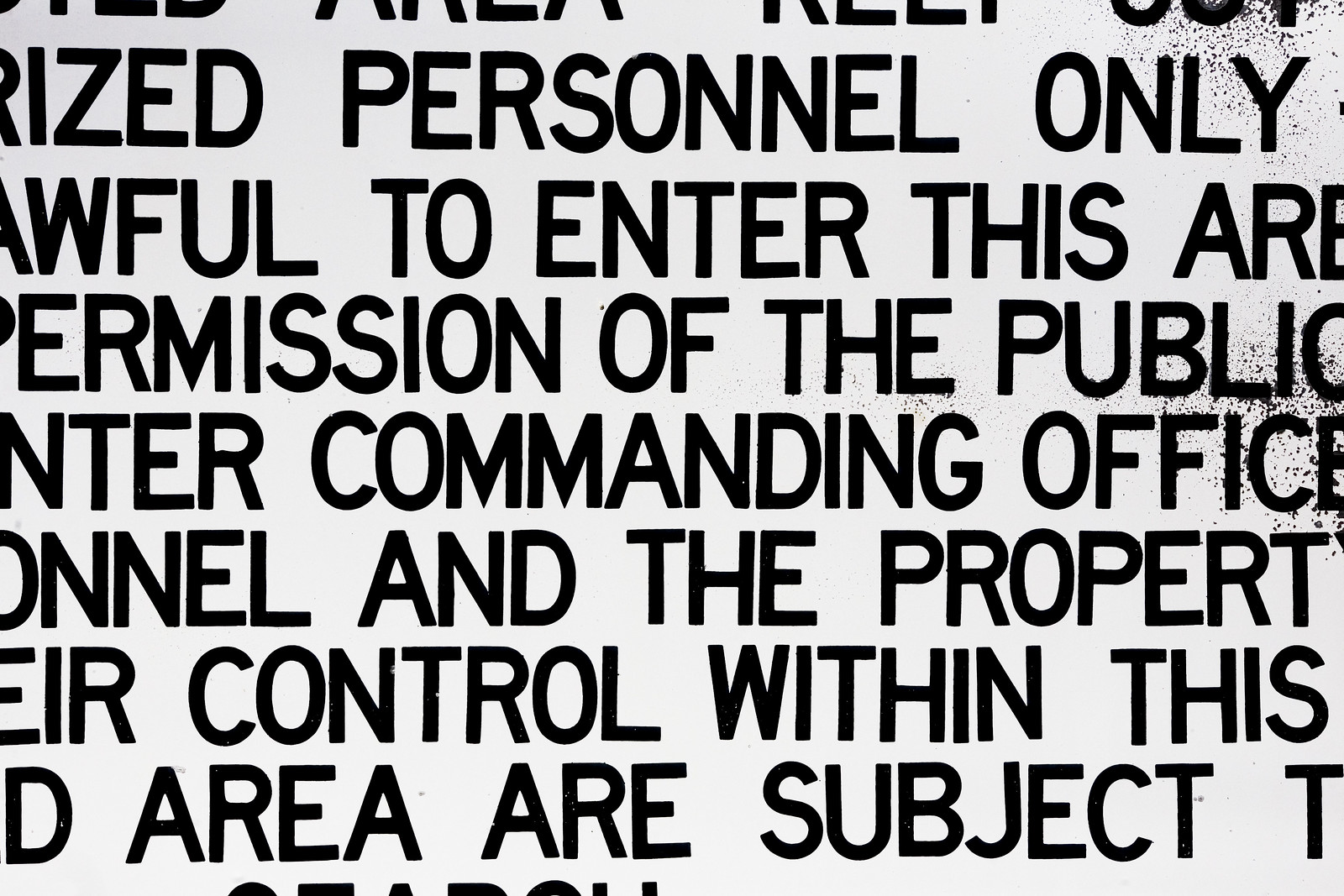This extreme close-up image captures a sign or piece of paper with black, fuzzy areas that suggest it may have been photocopied. The legible text, presented in large, block capital letters, includes partial phrases such as "personnel only," "awful to enter our," "permission of the public," and "inter commanding office." The message is fragmented, but mentions "proper air control within this area," and cuts off abruptly at the bottom. The text takes up the entire space from top to bottom and left to right, making it difficult to discern the complete message. The overall visual is characterized by the blurred, granular quality of the black text against a lighter background.